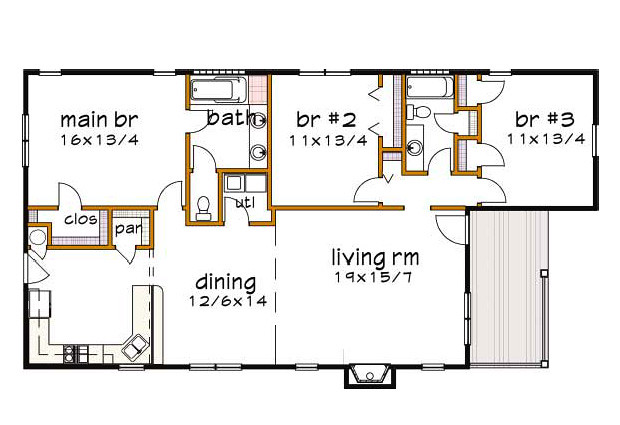This detailed rendering showcases a thoughtfully designed apartment layout featuring three spacious bedrooms and a combination of one and a half or potentially two full bathrooms. The main bedroom, situated in the upper left corner of the diagram, includes its own en-suite bathroom, offering privacy and convenience. Adjacent to the master bathroom lies a practical utility closet. The center of the home boasts a cozy dining room, seamlessly connecting to an expansive living room located to its right. Above the living space, the layout depicts two additional bedrooms—Bedroom Two positioned on the left and Bedroom Three on the right. These bedrooms share a well-placed communal bathroom nestled between them. Each room’s dimensions are clearly marked below their respective labels, providing precise measurements: the Main Bedroom measures 16 by 13 feet, while both Bedroom Two and Bedroom Three are each 11 by 13 feet. This comprehensive layout ensures a balanced blend of comfort and functionality.